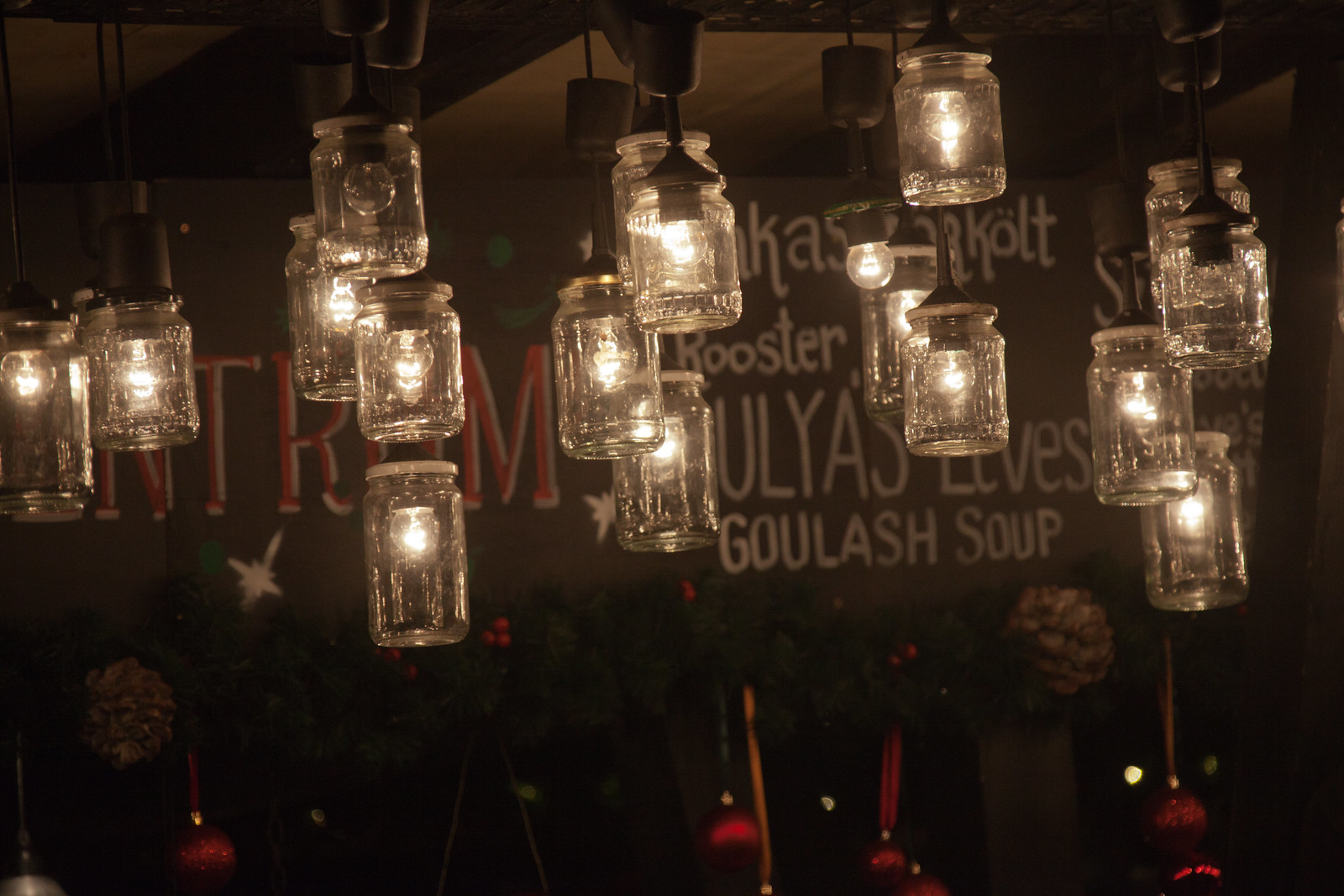The photograph captures the interior of a restaurant, showcasing an eclectic arrangement of ceiling lights fashioned from glass jars, reminiscent of mason jars, each encasing small circular light bulbs. About a dozen of these jar-lights hang from slender black poles affixed to a ceiling that appears to be a mix of black and gray hues. Amidst the warmly lit ambiance, several lights are notably unlit, with at least two exposed bulbs without jar covers and one plug devoid of a light fixture.

In the background, a chalkboard sign is partially obscured by the hanging lights. The readable text on the board includes the words "rooster" and "goulash soup" in white, with some additional text such as "lives" barely visible. Red text on the left side of the chalkboard is largely hidden, though the letter "M" is discernible. Below this sign, festive Christmas decorations adorn the space, including two pine cones—one on the left and another on the right—interspersed with red ornaments and possibly mistletoe-like greenery, evoking a holiday atmosphere. The overall scene is a cozy blend of rustic lighting and seasonal decor, suggestive of a warm and inviting dining environment.